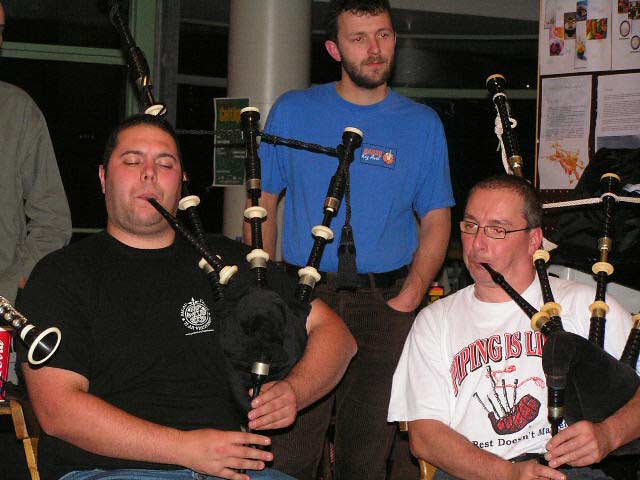In a cozy room with a window and bulletin board in the background, four men are captured in an engaging scene centered around music. In the foreground, two men are seated side by side, each deeply immersed in playing black bagpipes adorned with white and black pipes. The man on the left sports a black t-shirt showcasing a white emblem above his pocket, and has short black hair. His left hand securely grips the bagpipes. Beside him, to the right, is a man wearing a white t-shirt with red lettering that reads "Piping is Life." He also has short hair, small wire-rimmed glasses, and similarly wraps his left hand around his bagpipes. 

Standing between the two players in the background is a man attentively listening. He is dressed in a blue t-shirt and dark brown pants, with brown hair and a beard, his hands casually tucked into his pockets. 

Additionally, a barely visible fourth individual is present; only his arm in a green long-sleeved shirt can be seen, hinting at his presence in the scene. The demeanor and arrangement of these men suggest a moment of shared musical passion and camaraderie.